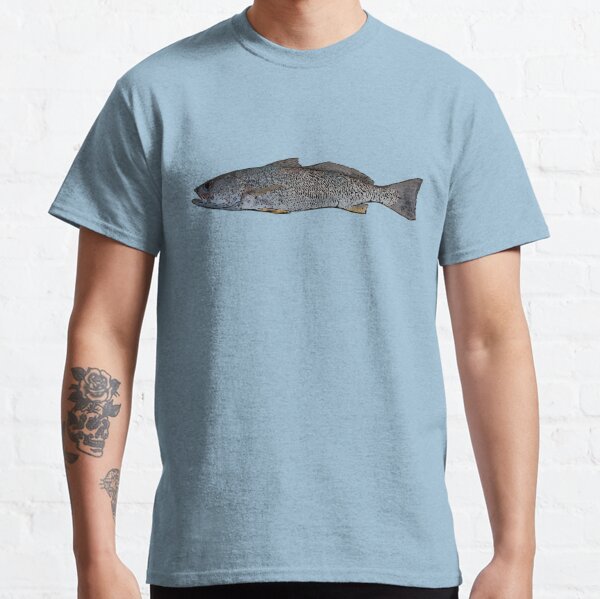This photograph features a man standing against a white brick wall. The image focuses on his upper body, capturing from his Adam’s apple down to a glimpse of his black pants. He is wearing a short-sleeve, light blue t-shirt adorned with a fish graphic on the chest area. This gray fish, viewed from the side, has its mouth open towards the left and is detailed with black spots and brown-tinged fins. His face is not visible, ensuring attention remains on the t-shirt and his tattoos. On his left arm, a dark tattoo depicting a skull with a rose above it is prominently featured, while additional tattoos can be seen on the inner part of his arm. The light source from the right side highlights his left arm and neck. His hands are not visible as they are placed underneath the t-shirt at his waist. The overall impression suggests the man might be modeling the t-shirt.